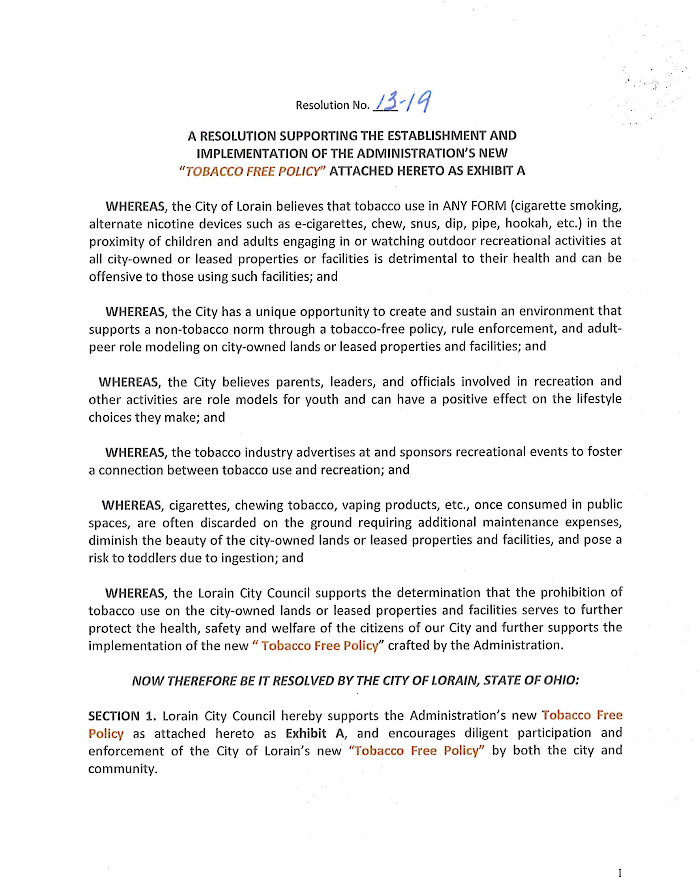The image depicts a formal resolution document titled "A Resolution Supporting the Establishment and Implementation of the Administration's New Tobacco-Free Policy, Attached Here to as Exhibit A." The resolution is from the city of Lorain, Ohio, and aims to prohibit the use of tobacco in all forms across city-owned or leased properties and facilities, highlighting a commitment to public health. The document begins with a handwritten resolution number "13-19" in blue ink. The title prominently features the term "tobacco-free policy" in brown font, emphasizing its significance. Multiple paragraphs follow, each starting with the bolded word "WHEREAS," outlining various rationales and stipulations of the policy. The bottom portion of the document contains italicized black text stating, "Now therefore be it resolved by the City of Lorain, State of Ohio," leading into Section 1 of the resolution. The structure suggests that more detailed provisions follow beyond the visible page.